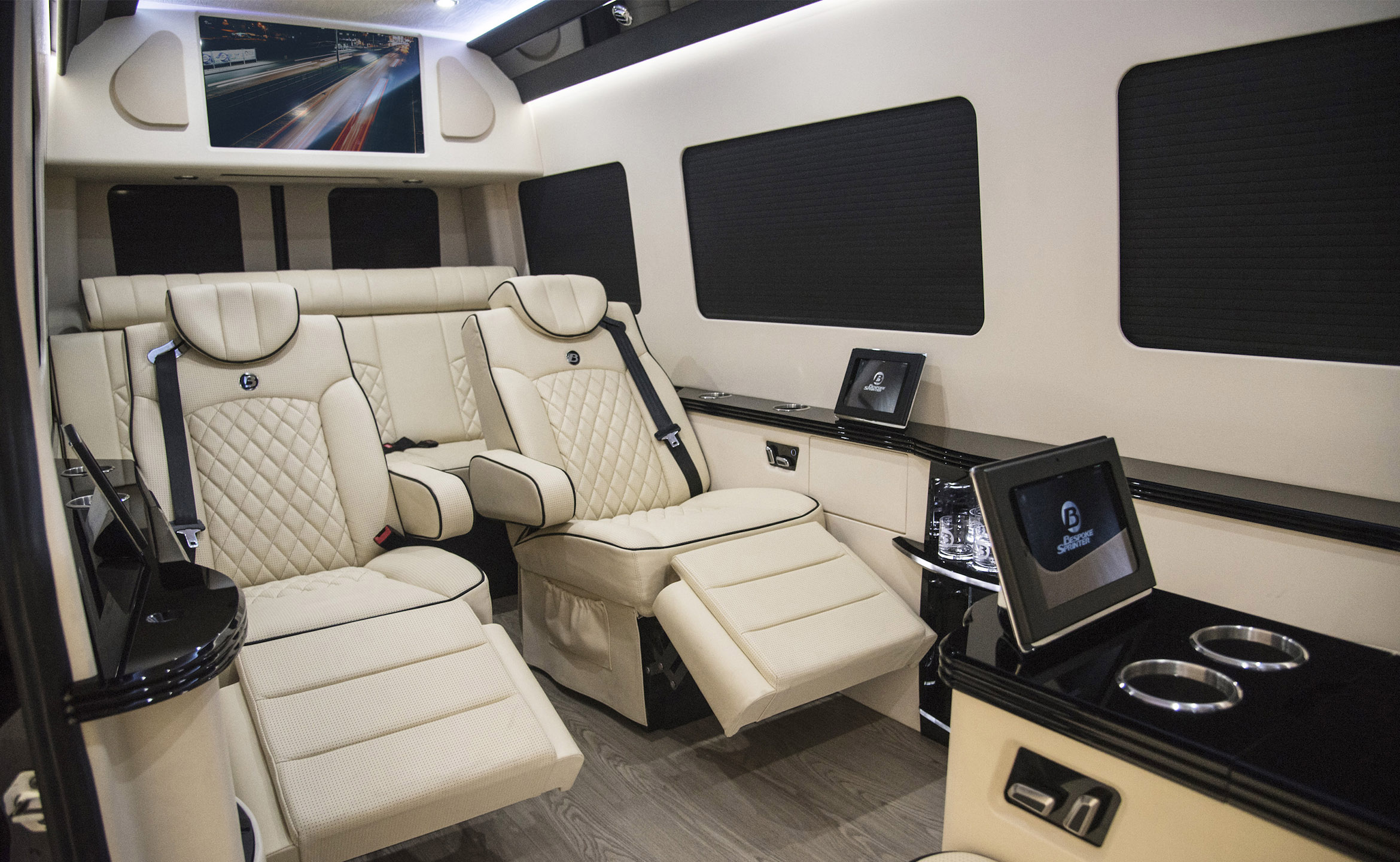This color photograph, taken in landscape orientation, captures the luxurious interior of a Sprinter van conversion, resembling a first-class airplane cabin due to its high-end features and spacious design. The interior is predominantly light cream, with quilted-stitched upholstery on two side-by-side reclining seats in the back portion of the van. Significant room and comfort replace the densely packed seating typical of economy setups. Behind these reclining seats is a versatile banquette cushion that converts into a bed. On the side rail, there is a ledge featuring a small screen, echoing the desk with another small screen situated in the front. The van also boasts a console with silver cupholders and seat controls, though these are partially out of view. A flat panel TV screen is mounted on the overhang in the rear, rotating to be visible from the front seats. The cabin is furnished with a wood laminate floor, and large rectangular windows wrap around the sides, allowing natural light to enhance the overall elegance of the space.